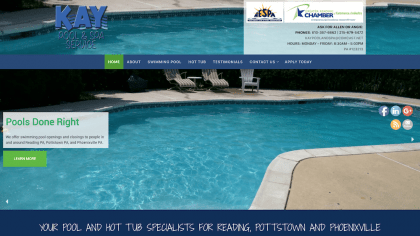This is the homepage for a pool construction business, identified as "K..." (with the rest of the name being unreadable). The page prominently features their tagline, "Pools Done Right," emphasizing their expertise in pool construction. The company serves the areas of Redding, Potsdam, Pottstown, and Finnville, specializing in both pools and hot tubs.

The navigation menu consists of seven tabs, including the home tab, although the details of the other six tabs are unreadable. The homepage also includes social media icons for their Facebook page, LinkedIn, Google Plus, and an unidentified orange icon, along with a user account icon.

The featured image on the page displays an inground pool that is beautiful with a unique, slightly curved shape. Surrounding the pool, there are three deck chairs positioned to the side, suggesting a relaxing spot for poolside leisure. The scene is set on a sunny day, enhancing the inviting atmosphere of the pool area.